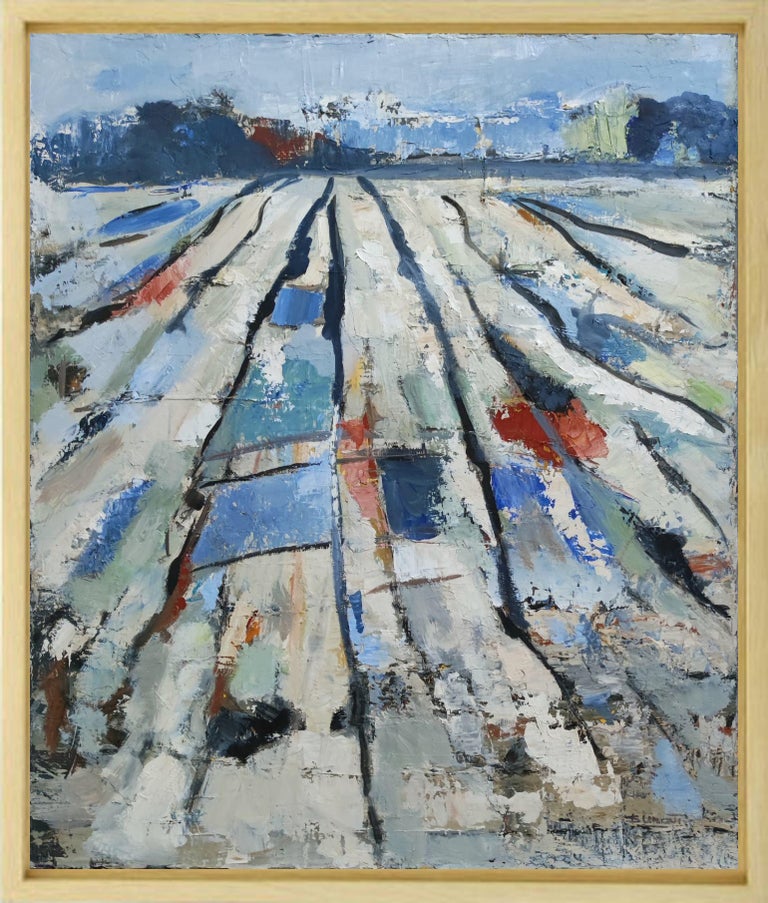This captivating watercolor painting, set within a light beige wooden frame, features an intricate abstract landscape that evokes a quilt-like texture. Dominated by vertical columns of varying colors—shades of white, gray, off-white, blue, red, yellow, green, and brown—the composition is intricately overlaid with dark blue and black lines. These lines create a patchwork mosaic that covers a significant portion of the piece, mimicking the appearance of abstract fields. In the background, dark blue mountains punctuate the horizon, some capped with white snow, all set against a bluish-gray sky. This complex interplay of colors and patterns guides the viewer's gaze from the detailed foreground to the serene mountainous backdrop, enveloping the scene in an almost icy, layered texture.